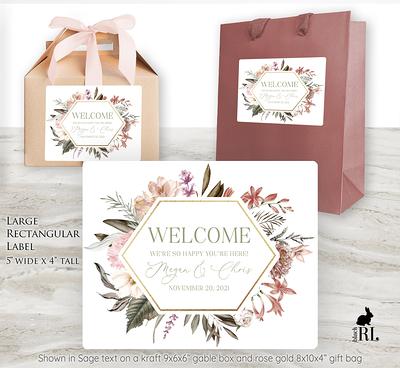This image is a digitally created advertisement showcasing various welcome bags. Set against a white wall backdrop and a gray marble tabletop, the top left features a light brown, box-shaped sack with built-in handles and a pink ribbon on top. Attached is a white hexagon-shaped sticker adorned with a floral pattern, bearing the word "Welcome". To its right, there's a maroon-colored gift bag also with handles and the same "Welcome" sticker. Below these bags, a white card is displayed prominently, detailing its size as 5 inches wide and 4 inches tall. The card, elaborately decorated with flowers and foliage surrounding the hexagon shape, is partially legible with a warm greeting and the date November 20th, 2021. An elegant handwritten name on the card is unfortunately faded. Additionally, the bottom right corner of the image features a logo of a black bunny with the initials "RL".